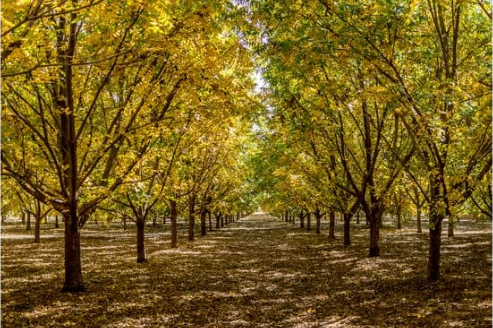The photograph captures a picturesque rural road that runs straight through the middle, blanketed by a thick layer of brown, dead leaves. This road is flanked on both sides by meticulously maintained trees, their trunks each six to seven inches in diameter, and adorned with a mix of gold and green leaves. These trees, seemingly planted with intention, form a natural canopy of interwoven leaves and branches overhead. The light gray sky peeks through the leafy cover, adding a soft, serene atmosphere. Extending beyond the trees that line the road, symmetrical rows and columns of identical trees stretch uniformly into the distance, creating a sense of endless order and tranquility in this bucolic setting.